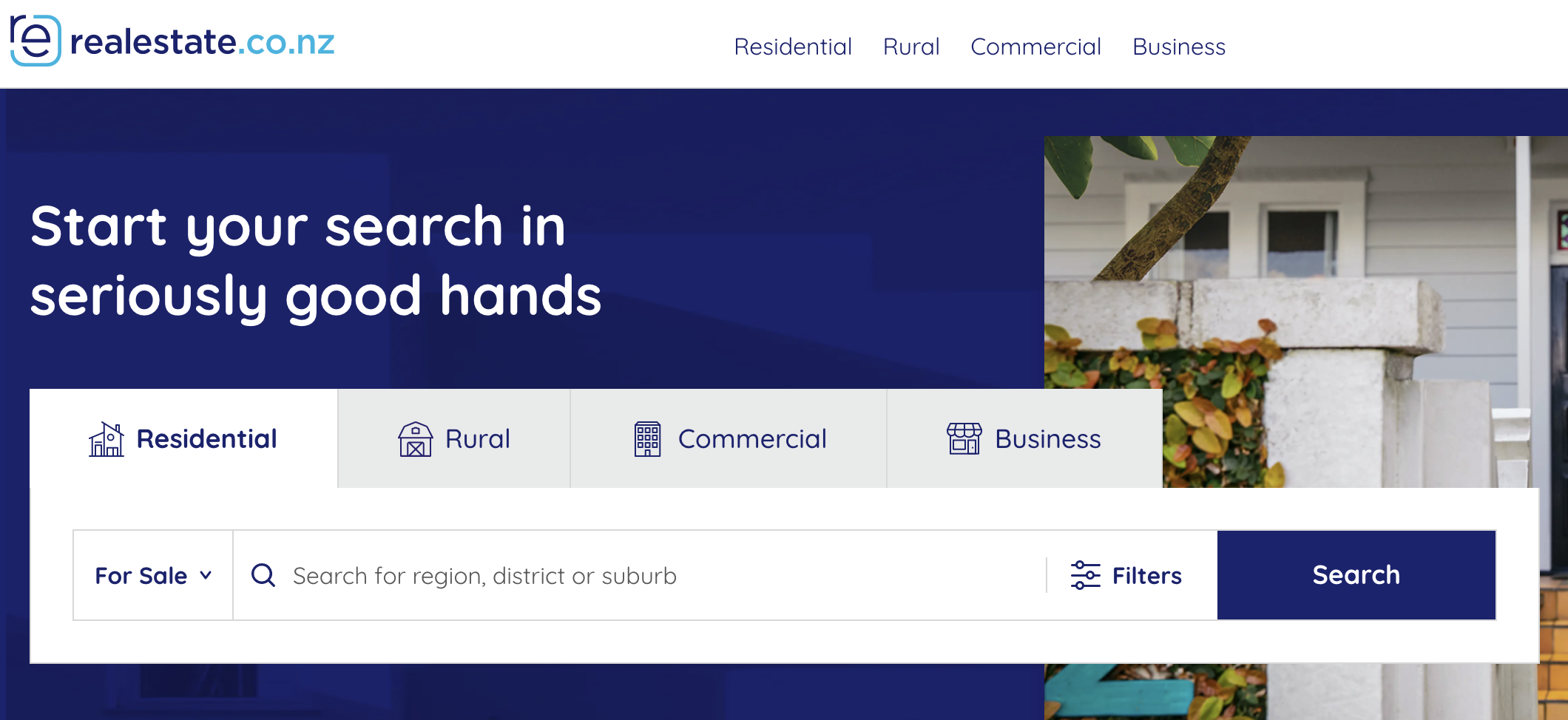This is a detailed screenshot of the homepage of the real estate website, realestate.co.nz, which caters to property listings in New Zealand. At the top of the page, the main navigation menu offers tabs for different property types, including Residential, Rural, Commercial, and Business. Below this menu, a dropdown filter allows users to select properties that are For Sale, For Rent, or other options. 

The central search bar invites users to "search for region, district, or a suburb," with additional filter options available for more tailored searches. A prominent blue button labeled "Search" stands out, encouraging users to initiate their property search.

A banner across the website carries the slogan, "Start your search in seriously good hands," instilling confidence in potential users. Below the banner, an image features a house or a related structure, adding a visual appeal to the page.

The logo of realestate.co.nz is distinctly placed in the top left-hand corner. It consists of an "R" positioned above an "E," both framed by a blue box that extends from the bottom of the "R" to the top, wrapping around the "E," creating a stylish and memorable emblem.

The design and layout of the website suggest that it caters to various kinds of property searches—whether for residential homes, rural areas, commercial buildings, or business opportunities, offering a comprehensive platform for users looking to explore different types of real estate across New Zealand.